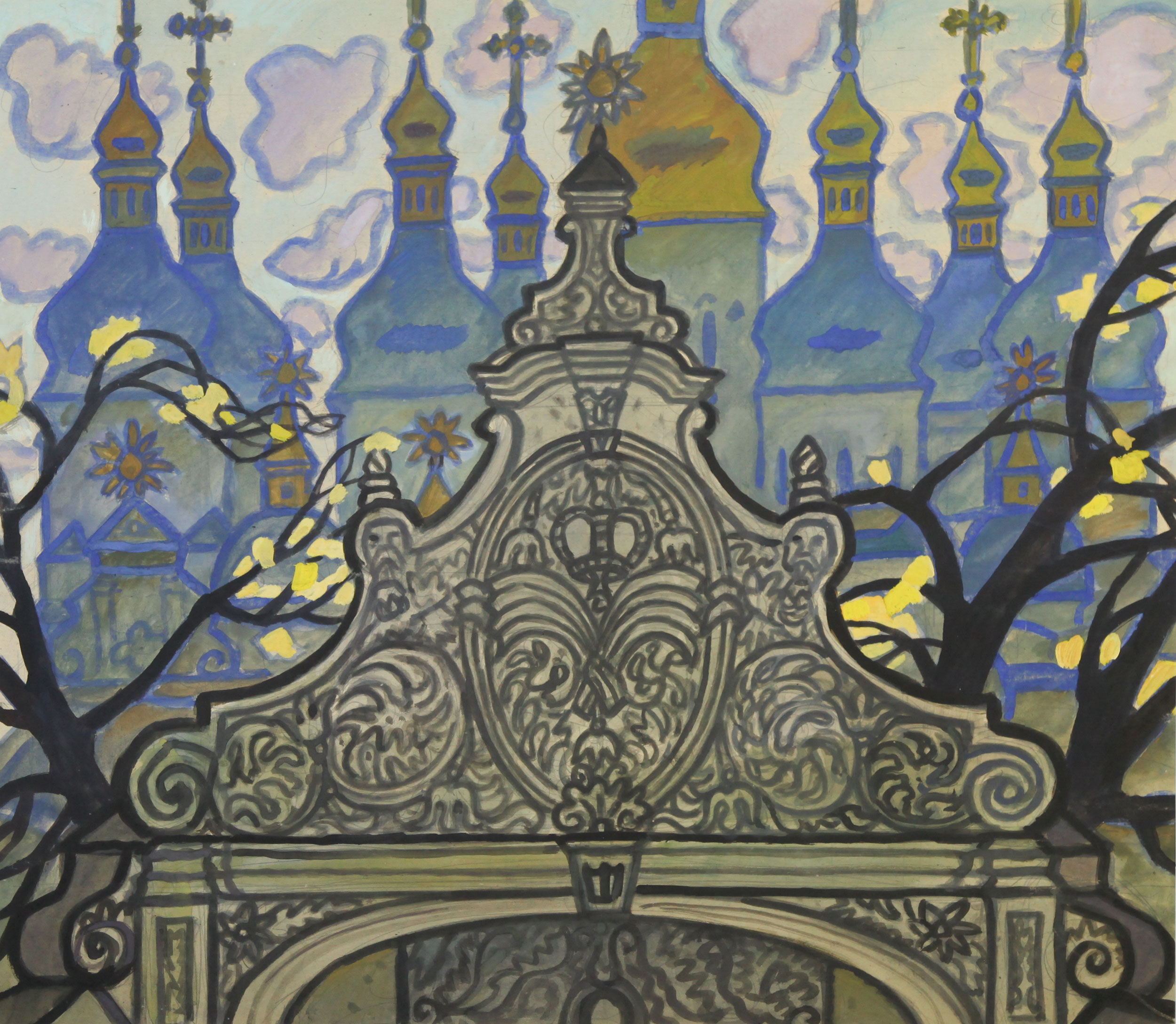The image depicts a painting titled "Zaborsky Gate" by a Ukrainian painter. Dominating the foreground is the top of a very ornate gate, reminiscent of a throne or intricate chair, adorned with circles, drawings, and possibly faces, and culminating in a flower-like design. This central structure, rendered in shades of brown and gold, features a stained glass effect and exudes an air of ornate splendor. To its right and left stand bare-branched trees.

In the background, a succession of towers appears, resembling Byzantine-style architecture or the onion domes of St. Petersburg, Russia. These buildings, evocative of Coke bottles, display a mix of blue and gold, with each steeple topped by a golden cone or cross. The backdrop suggests a sky tinged with light yellow, hints of blue, and small, crudely drawn pink and orange clouds outlined in a bluish-purple hue. The overall composition has a watercolor-like, somewhat muddy aesthetic, adding to its unique charm and intricate detailing.